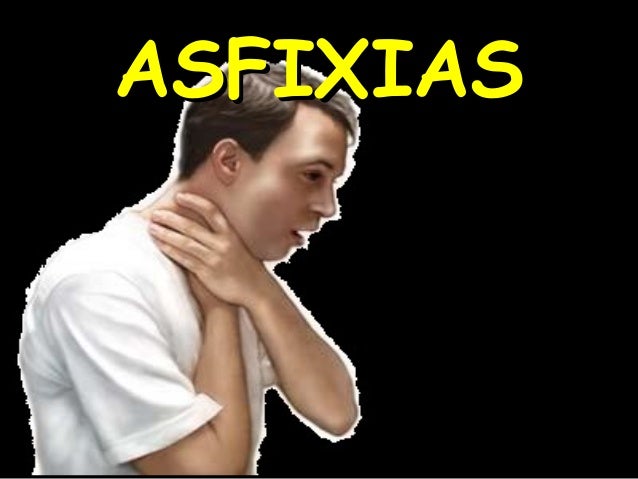In this image, a young Caucasian man is shown against a completely pitch-black background. The scene appears photoshopped, with a noticeable white border around the man's profile, which is facing the right side of the image. He has short, combed-over brown hair and wears a white t-shirt. His expression is intense, with his mouth slightly open and his head tilted forward, gazing slightly downward. He grasps his neck with both hands as if choking himself, his arms crossed. Positioned on the left side of the image, the man is depicted with stark clarity. Dominating the top of the image, bright yellow capital letters spell out "ASFIXIAS." The overall composition uses a color palette primarily consisting of black, white, yellow, brown, and tan.